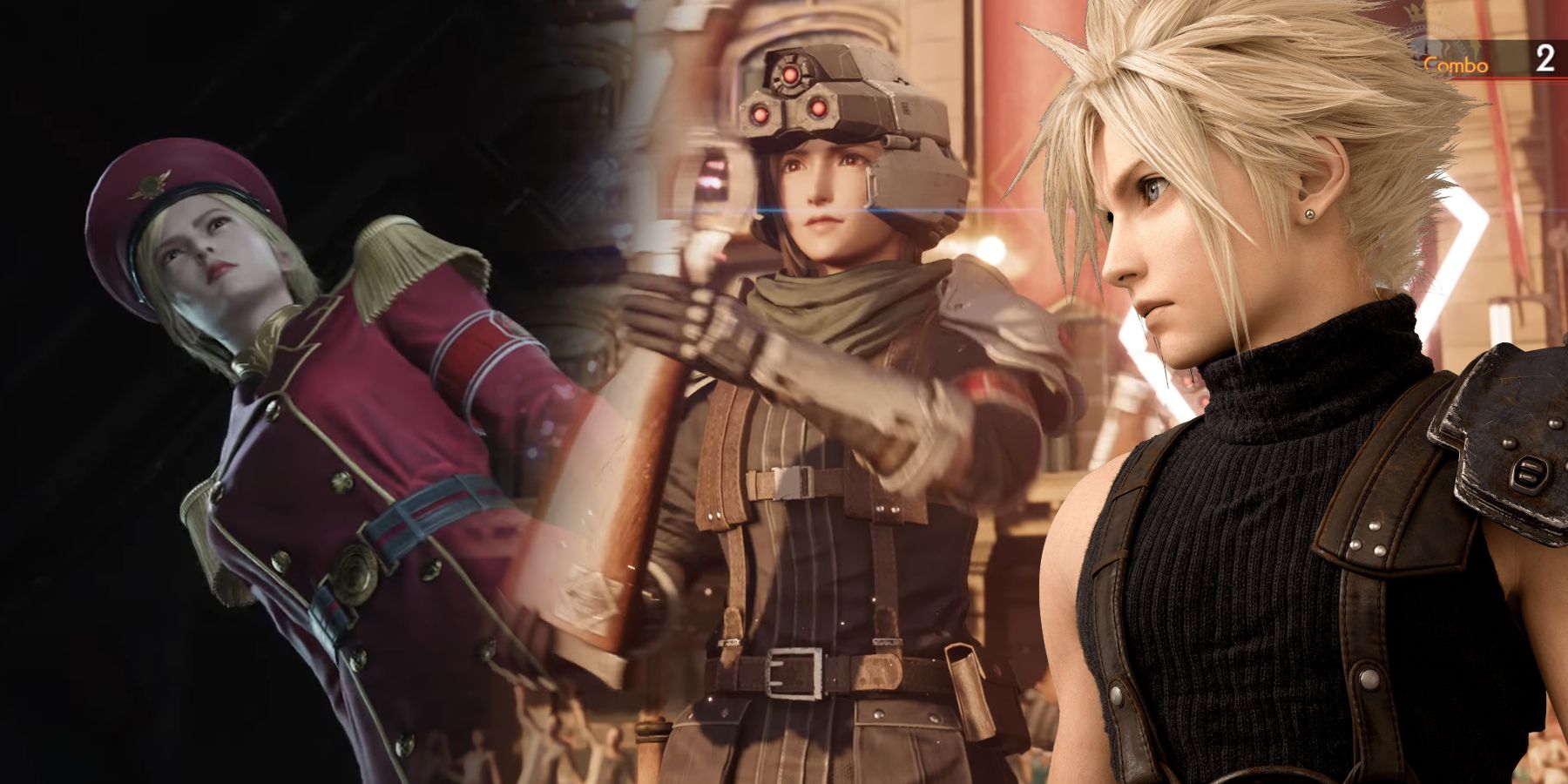This is a still from a video game, possibly Final Fantasy 7 Remake, featuring three different images of a blonde woman, likely the same character, dressed in various outfits that suggest a military or combat theme. On the left, the image is shot from a low angle, showcasing the woman in a maroon soldier's uniform with gold epaulets, a black belt with a prominent gold buckle, and a matching red hat resembling an Air Force cap. She also has short hair. The middle image features her in a rugged brown military outfit, equipped with padding on her shoulders, gloves, and what appears to be a rifle in her hand. She looks ready for combat with added protective gear, including a gadget on her head for magnification. The last image on the right shows a side profile of the same woman in a black, sleeveless turtleneck. Her spiky hair, earring, and shoulder padding are visible, along with straps across her torso, suggesting the presence of a weapon or gear strapped to her back. All three scenes underline her combat-ready appearance with varying uniforms and accessories.